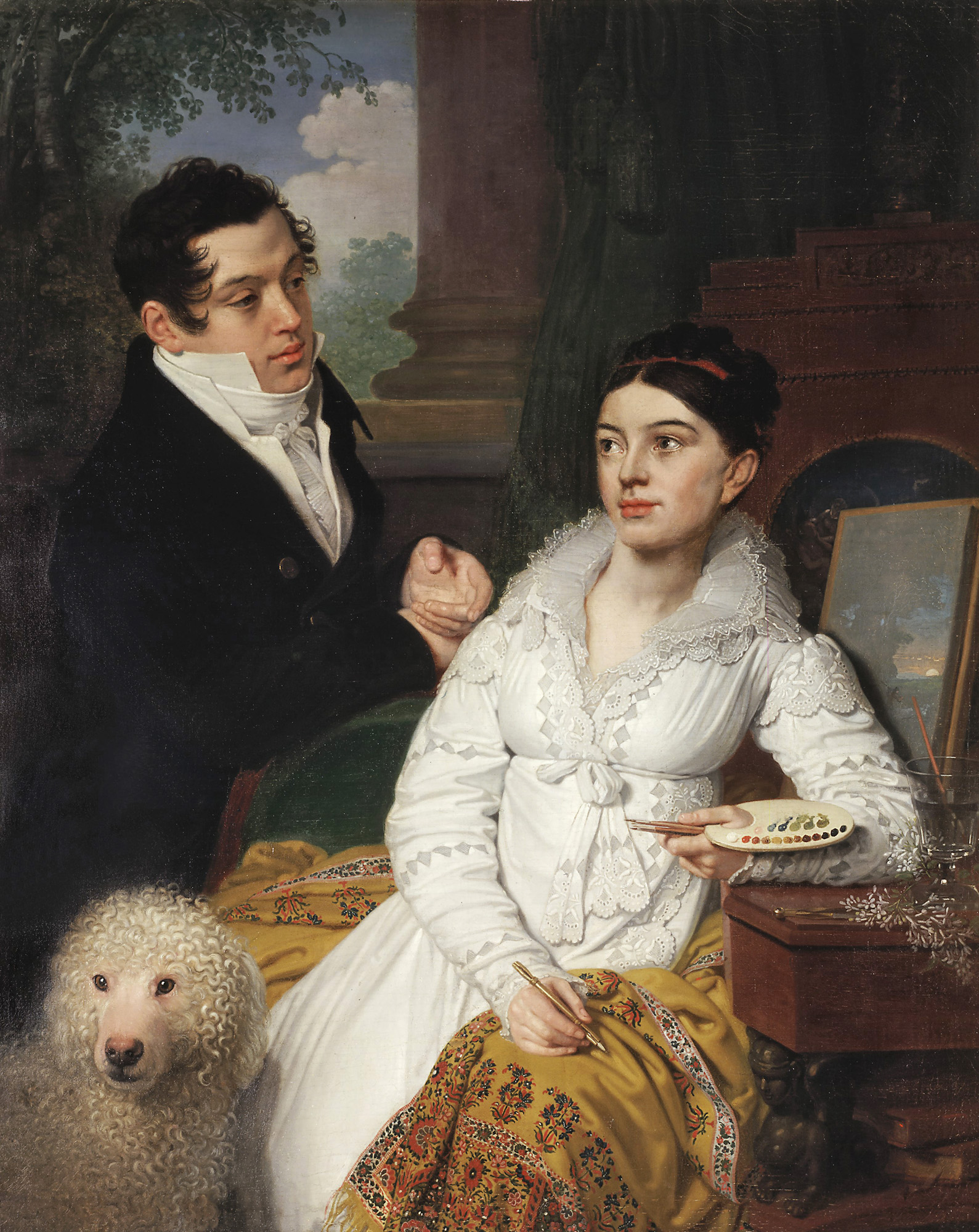This Victorian-style painting captures a serene outdoor scene, potentially at the entrance of a mansion, with a backdrop featuring a brown column, steps, trees, a blue sky, and white clouds. In the foreground, a woman in a green chair commands attention. She's adorned in a white, lacy dress with a red bow in her black hair, which is tied up. She holds a small easel with her thumb through its hole, displaying blobs of paint, and a gold paintbrush in her other hand. A yellow or gold blanket drapes over her chair. Resting on a wooden side table next to her, also holding some paintbrushes, is a glass of water. Adjacent to her, a white curly-furred sheepdog with dark eyes gazes straight ahead. Leaning towards her is a man dressed in a black coat and a white shirt with a high, turned-up collar that reaches his cheekbones. He has black, slightly tousled hair. Both figures have fair skin and red lips, contributing to their striking presence in the painting.